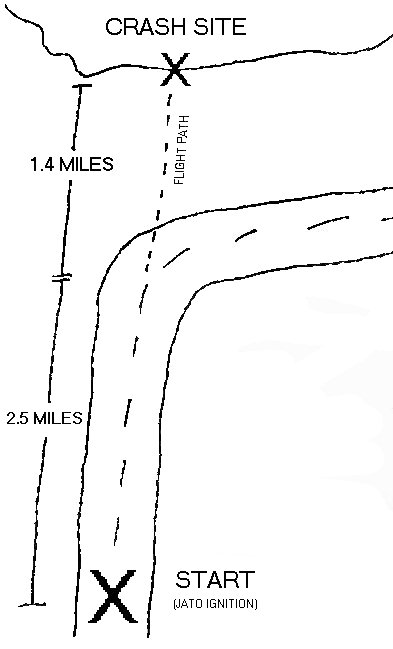The black and white image depicts a crudely hand-drawn map highlighting the path and impact site of an unspecified accident. At the top, the label "CRASH SITE" is written in bold black font, with an 'X' marking the precise location. Below this, the term "FLIGHT PATH" is noted, suggesting the trajectory of a vehicle, possibly an aircraft. A dotted line representing this flight path continues straight along a road that curves to the right, indicating where the vehicle failed to follow the road and continued straight to the crash site. At the bottom of the image, another 'X' is labeled “START,” with "JATO IGNITION" inscribed beneath it, marking the journey's initiation point. The road in the image is depicted as a two-lane route with a dotted centerline, moving from the bottom center upward before curving right. Along the left side of the map, mile markers are displayed at 2.5 miles and 1.4 miles, denoting distances from the starting point to various positions on the map. The overall impression is that of a rudimentary illustration detailing the sequence and distances involved in an accident scenario.